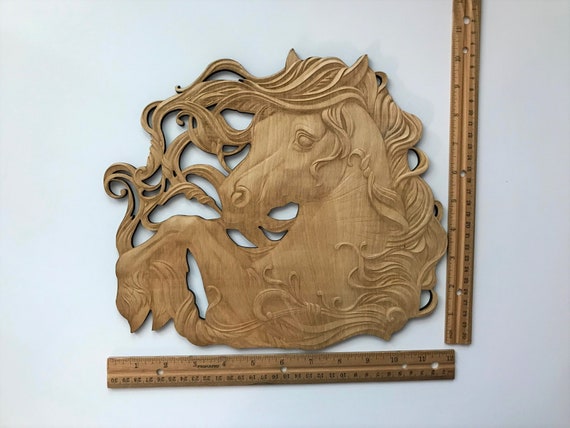This image features a striking carving of a horse, possibly crafted from wood or metal, in a light tan, sandy brown color. The detailed design, meant to be mounted on a wall as a decorative placard, depicts the horse rearing up on its hind legs with its two front hooves in the air. The horse's head is turned to face the viewer, highlighting its expressive eyes and long, flowing, curly mane, which is the primary focus of the artwork and wraps around the horse's neck and legs. The background is stark white, accentuating the carving's intricate details, including some darker areas on the mane that suggest either an unfinished texture or deliberate shading for emphasis. To provide a sense of scale, rulers are placed along the bottom and right side of the sculpture, indicating that the artwork is approximately a foot in length and height.